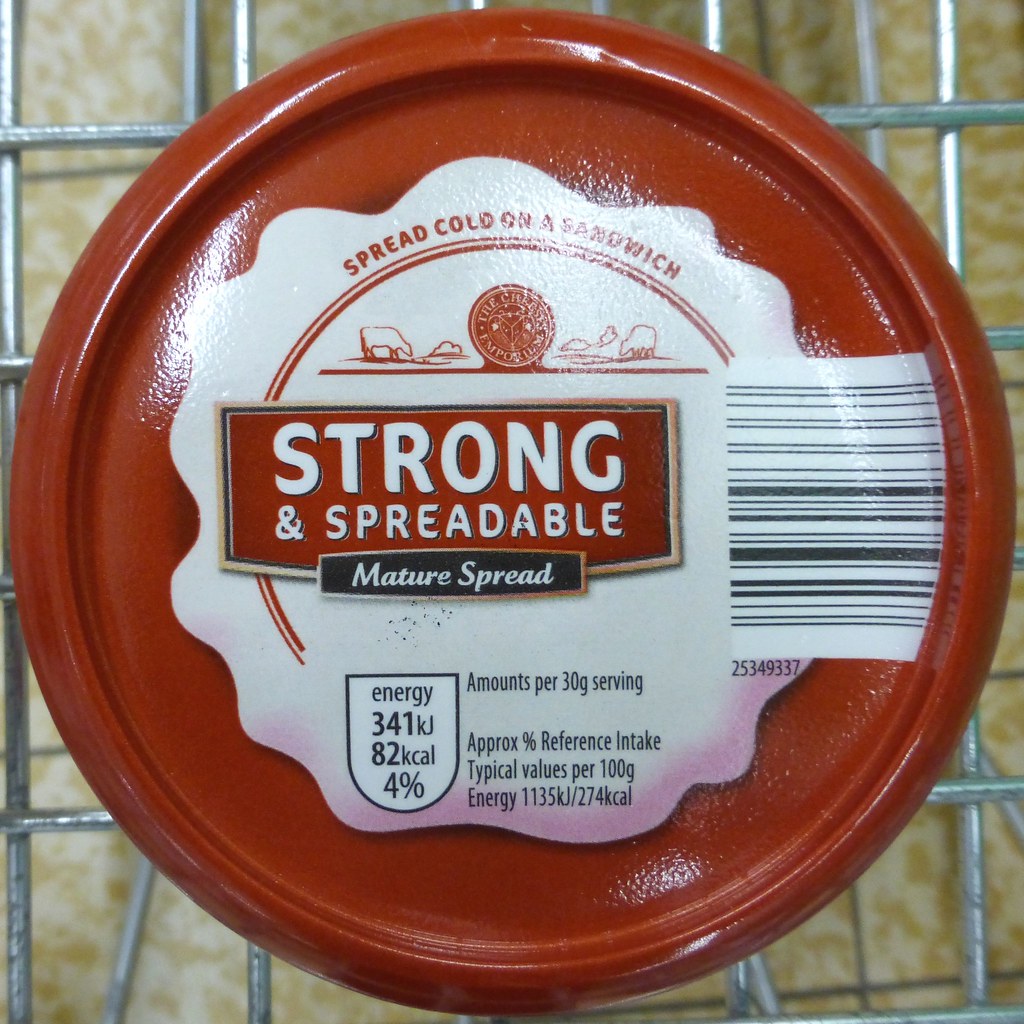This color photograph is a detailed close-up of a circular grocery item sitting in a wire metal shopping basket, viewed from the top down. The item is most likely a tub of butter or a similar spread. The lid features a burnt orange background with a white splat-like image serving as the backdrop for the printed text. Prominently displayed in bold letters, the text reads "Strong and Spreadable." Below that, in a red badge, it says, "Mature Spread." Additional instructions state to "Spread cold on sandwich." The label also provides nutritional information, indicating amounts per 30-gram serving: Energy 341 kJ, 82 kcal, 4%. It further details the approximate percentage reference intake and typical values per 100 grams: Energy 1135 kJ / 274 kcal. The packaging also includes a barcode.